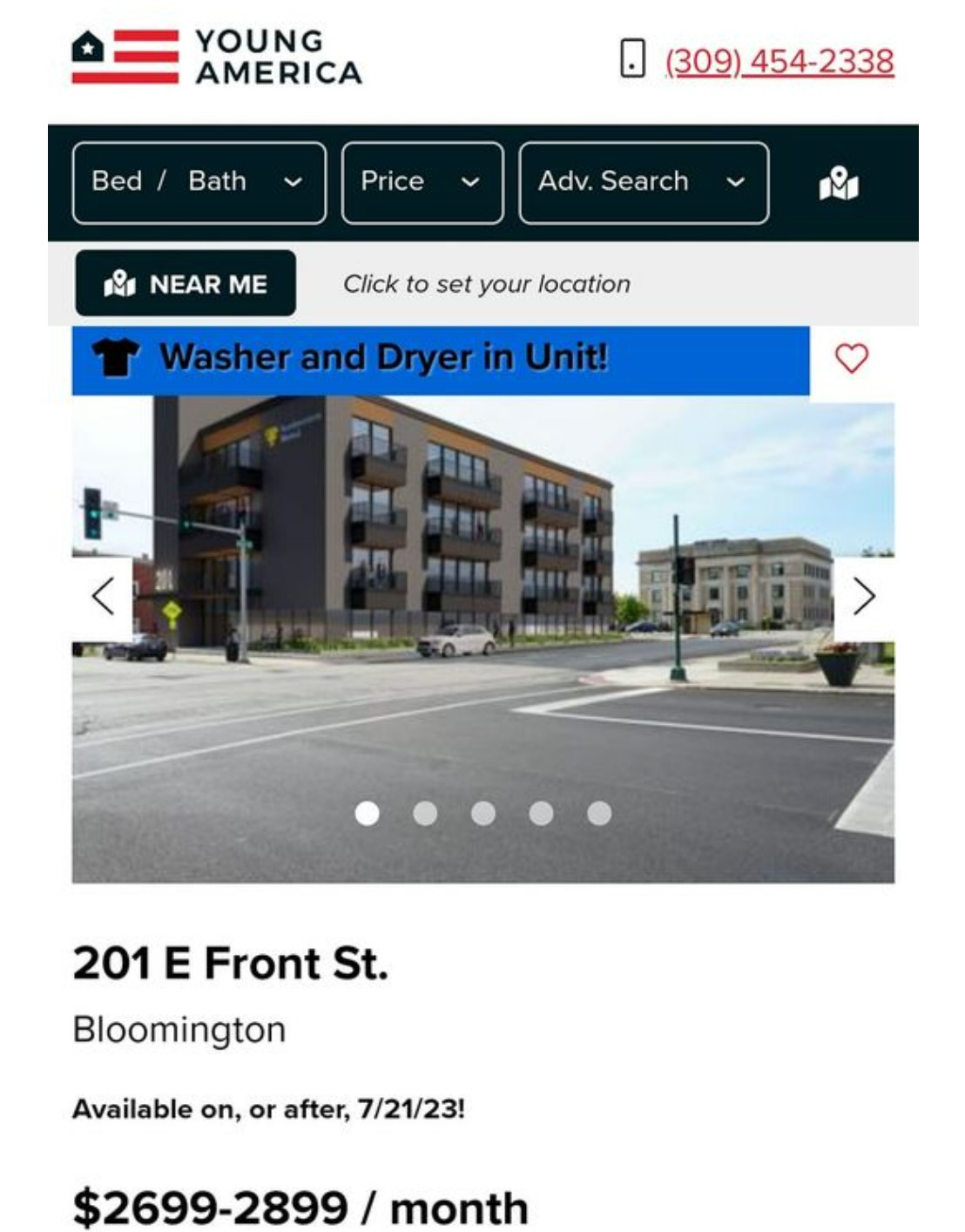**Detailed descriptive caption:**

This detailed screenshot, captured on a mobile device, showcases an app designed for finding apartments. Prominently featured in the top banner is the app or website logo and a unique emblem for "Young America." The emblem cleverly incorporates an American flag motif with houses replacing the stars in the upper left-hand quadrant. Adjacent to this, on the right-hand side, the company's contact number, 309-454-2338, is displayed.

Moving down the screen, we see an array of search filters used by the user, which include options to filter apartments by bed and bath count, price range, and an advanced search feature. This section also includes a map icon, indicative of additional search functionalities. Directly below these filters, another button adorned with the same map icon reads "Near Me" and prompts users to "Click to Set Your Location."

The centerpiece of the screenshot is a vivid photograph of the available apartment, accompanied by a note that highlights the inclusion of an in-unit washer and dryer. The image depicts a standard American street corner, with the view directed towards an opposing corner where the apartment complex stands. The building itself boasts a modern design with gray and dark brown coloration. The accompanying text provides crucial details, listing the address as 201 East Front Street, Bloomington, and noting the rental price range of $26.99 to $28.99 per month.